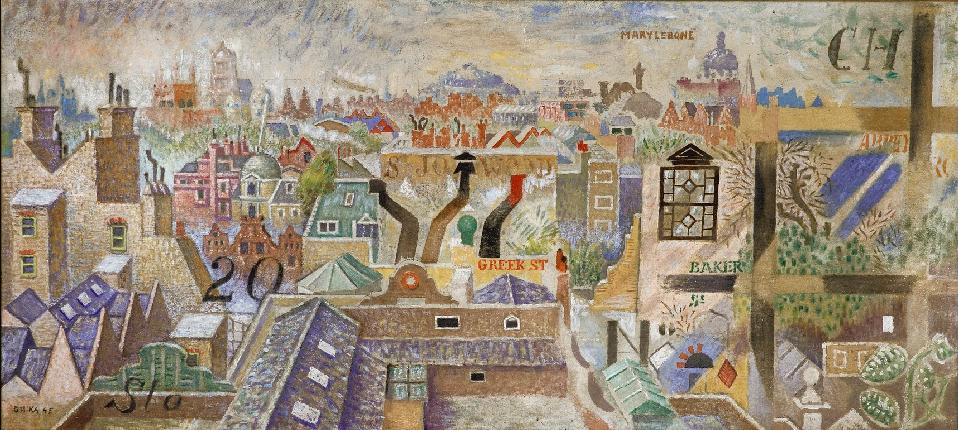This is a colorful oil painting titled "London Roofs" by artist Nikos Hadziakiriakos-Gikas, created circa 1945 in a Cubist style. The landscape-oriented artwork provides an overhead view of a densely packed cityscape with a myriad of buildings in various colors such as green, blue, gray, brown, red, orange, and a standout entirely pink building. Number "20" is marked on a building in the bottom left corner, and street labels including "Greek St" in bold red letters and "Baker" can be discerned on certain structures. The scene is framed by a vibrant sky and includes notable details like rock towers, gray tile roofs, a courtyard in the front center, dark brown paths, a brown tree trunk, a blue pond, and a dome-shaped building in the top right. The bottom of the image features the letters "S-L-O" in black, and an artist’s signature is also visible in the bottom left. Overall, the painting captures a vivid, intricate depiction of the city with buildings extending as far as the eye can see.